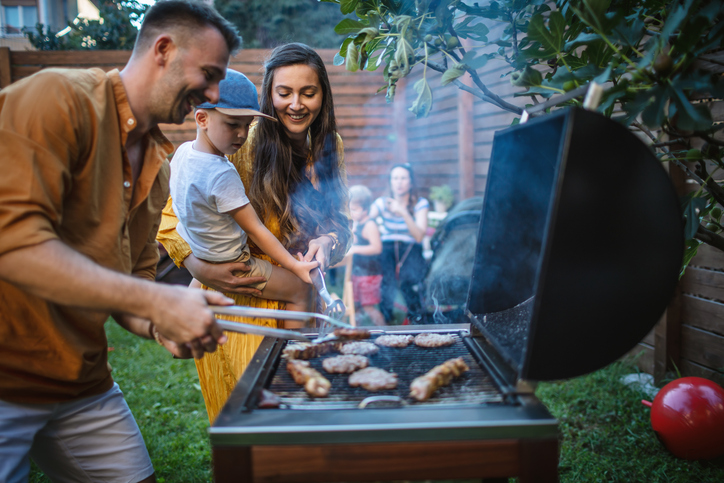This horizontally aligned rectangular photograph captures a vibrant backyard barbecue family gathering. Central to the image is a man in a tan button-down collared shirt and khaki shorts, leaning over a brown barbecue grill with black and silver handles. He is holding silver tongs, poised to flip a juicy burger amid the smoke wafting up from the grill. On the grill, there are about 8 to 10 burger patties and a couple of kebabs sizzling away. Beside him, a woman with long, straight brown hair, wearing a gold dress, holds a young boy around five years old who is donning a baseball cap, a short-sleeved t-shirt, and shorts. Both the man and woman are smiling down at the food, while the boy observes curiously.

In the background, several guests or family members are seated, enjoying the sunny day. They are positioned near a medium-colored wooden fence made of horizontal slats, which appears to be about 8 feet tall. The lush green lawn features a large ball, hinting at playful activities. Additionally, a bush or tree extends over the grill area, adding a touch of greenery to the lively scene.